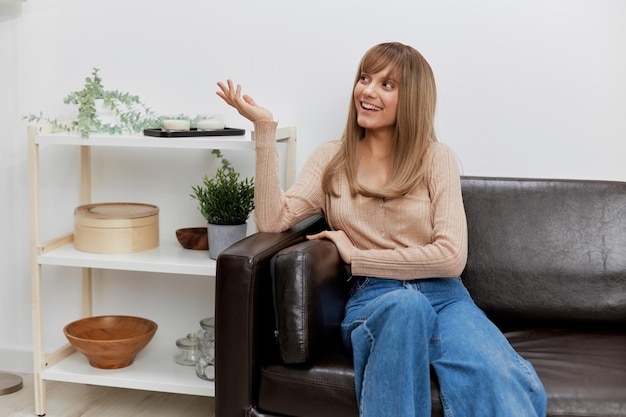In a bright, airy room with plain white walls and pale wood floors, a young woman with long, dirty blonde hair and bangs sits on a dark brown leather couch. She is dressed in a beige, long-sleeve sweater and blue, wide-leg jeans. Her elbow rests on the arm of the couch, and her hand is pointed outward, indicating she might be in the middle of a pleasant conversation or reminiscing fondly. The couch, reminiscent of one found in a psychiatrist's office, is positioned to the right side of the photo, partially out of view. Next to the couch is a three-tiered shelf made of white and possibly bamboo or light pine wood. The top shelf holds a black dish with coasters and a pale green plant. The middle shelf contains several glass dishes, a lighter brown hat box-type container, and another plant. The bottom shelf features a brown pottery bowl alongside some glass jars. The room’s minimalistic decor enhances the soothing and reflective atmosphere, highlighting the woman’s expressive smile as she gazes to the left.